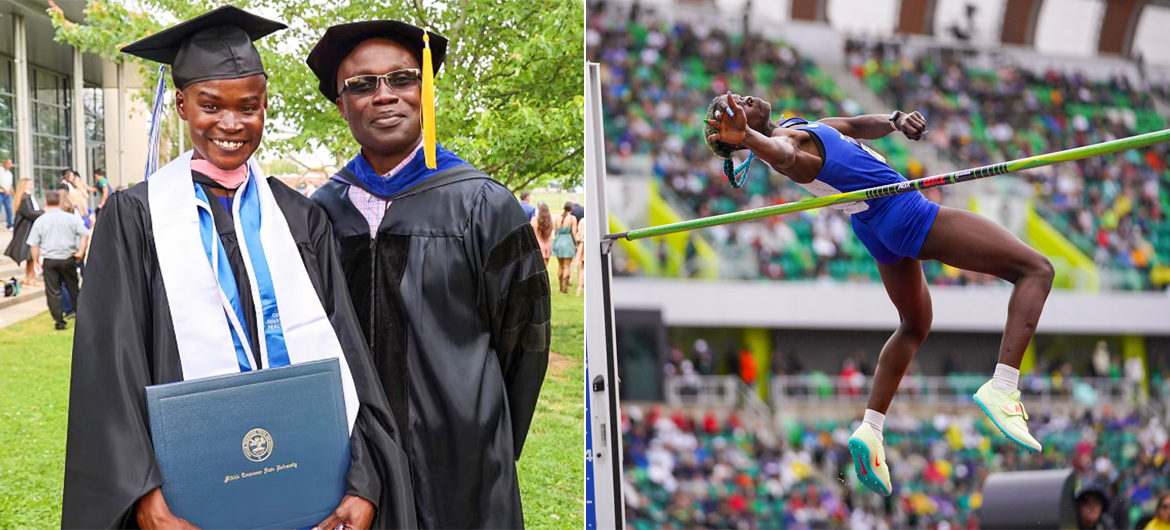This horizontal composite color image showcases two side-by-side photographs. On the left, a young woman and an older man are celebrating a graduation ceremony. The young woman, likely the student who has just graduated, is wearing a black graduation cap and gown, with a white and blue striped stole around her neck. Her tassel is blue and white, possibly indicating school colors. She proudly holds a diploma in her hand. The older man beside her, possibly a professor or a proud father, is wearing a similar black cap with a yellow tassel, skinny rectangular glasses, and a blue stole draped around his neck and trailing down his back. They stand in front of what appears to be a college campus.

On the right-hand side, the same young woman is captured mid-air, performing a high jump at a sporting event. She is dressed in a blue and white sports uniform and wears cream and aqua-colored Nike sneakers. She's vaulting backwards over a horizontal green pole, reaching back with her right hand. The background is blurred, but it's apparent there's a large crowd in the stands, largely dressed in green, suggesting school colors or a themed event. This juxtaposition of images highlights her exceptional achievements both in academics and athletics.